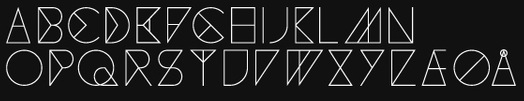A high-quality screen capture showcases a large black rectangle filled with abstract, white alphabet-like symbols. The characters appear distinctly coded and artistic. Each symbol is unique: the 'A' resembles a triangle, the 'B' maintains a traditional form, the 'C' curves like a crescent moon, and the 'D' features a triangle within it. The 'E' consists of several small triangles, giving it a fragmented appearance. Both 'M' and 'N' look conventional, as does the 'O'. However, the 'P' is distinctly triangular. Some of the letters possess a cursive flair, enhancing their unusual and abstract design. The black rectangle that hosts these characters is sharp and clear, free of blurring or pixelation, with no additional images, such as people, animals, or objects. There are two rows of these symbols, with the last character in the second row resembling a pyramid with a circle atop it. Overall, this image is solely focused on the intriguing typographic designs, inviting viewers to interpret the abstract forms.